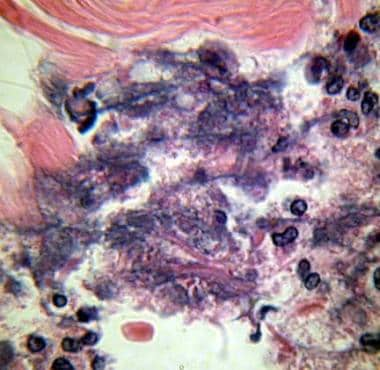This image, possibly an abstract painting or a close-up view of a substance under a microscope, is a smaller square picture with no border or text. It features a swirl of pink and tan hues extending from the top left to the right side. Interspersed within this swirl, particularly on the upper right, are clusters of small, raisin-like shapes, potentially resembling blueberries, numbering around six or seven. These shapes are also scattered down the middle and densely grouped in the lower left corner.

Below the pink and tan swirl, the central area transitions into a mix dominated by white, interwoven with purplish-black tones. The right side prominently displays these purple and white colors, along with additional small, raisin-like shapes, which continue to appear throughout the image. Towards the bottom center, the palette shifts primarily to white, accented by a small chunk of circular pink area. This intricate and colorful composition, with its blend of pink, white, and various shades of purple, creates a visually engaging scene, textured with small, dark clusters that add to its abstract and detailed nature.